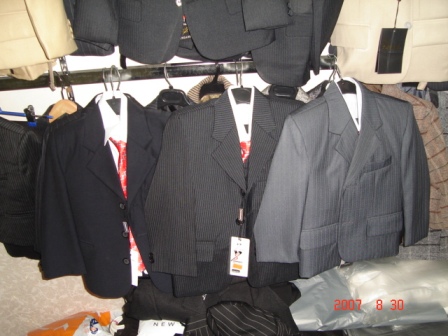This photograph, likely taken in a store, showcases a selection of children's or small-stature suits meticulously arranged on black hangers suspended from a metal rod. Dominating the scene are three prominent suits. The one on the left features a black jacket paired with a white button-up shirt and a red tie adorned with white triangle patterns. The central suit, possibly dark gray or black, is distinguished by white stripes and similarly paired with a white shirt and red tie. To the right, a dark gray suit with wider white stripes complements the lineup, though its red tie is not visible. The suits, which vary in texture and design, include patterns such as solid colors and different shades of gray. Additionally, the background reveals more suits hanging above and behind the front display, including a tan and an off-white suit on the right and what appears to be a brown plaid suit. An orange plastic bag is noticeable on the left, while a plastic covering encases part of the central suit. A red date stamp in the bottom right corner reads "2007 8 30," subtly indicating the image's capture date.